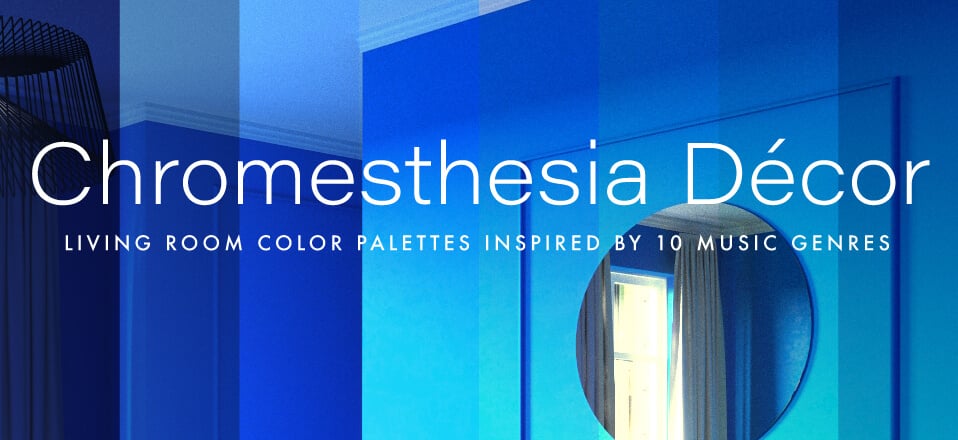The image showcases a promotional photograph for Chromesthesia Decor, featuring the text "Chromesthesia Decor" prominently in white lettering, with the subtitle "Living Room Color Palettes Inspired by 10 Music Genres" just below. The room depicted is a study in gradient blues, starting with a dark navy blue on the left and transitioning to a lighter ocean blue on the right, representing various music genres through color. The walls, while primarily blue, become lighter as they approach the room's corner and are capped with white above the crown molding. A round mirror is positioned to reflect a blue-edged window with sunlight streaming in through the curtains. Additional room details include the visible crown molding and part of a lamp, creating a cohesive space that illustrates the gradual shift in hues and artistic inspiration drawn from music.